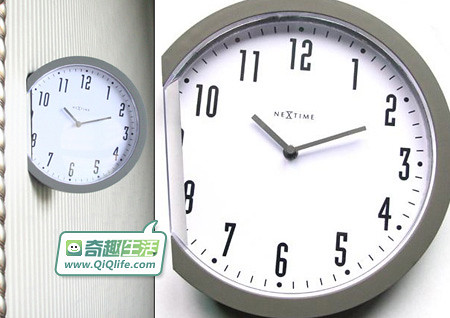The image is a composite consisting of two horizontally aligned sections. The left section features a wall clock partially embedded into a striped, vertically-oriented wall. The clock is lodged into the wall from the 8 o'clock to the 10 o'clock position, giving the impression that it has been forcefully inserted or thrown. This section is narrower compared to the right section.

The right section provides a close-up view of the same clock, detailing its gray bezel and the white clock face. The hour and minute hands are also gray, and the numerals around the perimeter of the clock face are arranged from 12 to 11 in a standard format. The brand name "NEXTIME" is clearly visible on the clock face. Additionally, in the lower left corner of this section, there is a green, quotation-styled rectangle containing a small figure and some characters resembling those from an Oriental script. Below this, the URL "www.qiqlife.com" is displayed.